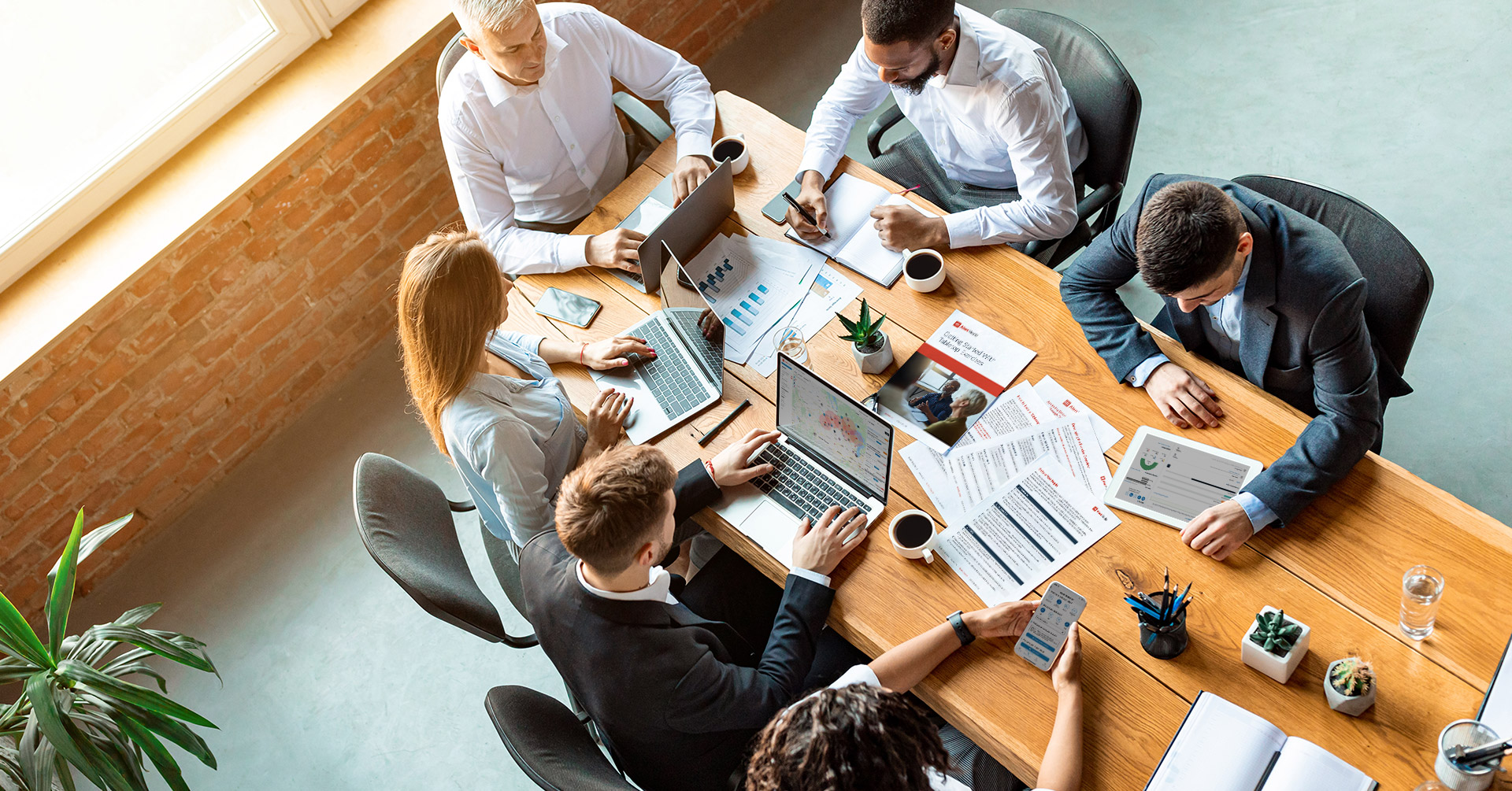This aerial photograph captures a detailed view of a professional business meeting taking place around a long, beautifully finished wooden table composed of three wide planks. The group consists of five individuals—two females and three males—all dressed in formal business attire including dress shirts, ties, and some wearing suit jackets, emphasizing their professionalism. At the table, three individuals are engrossed in their laptops while one person is writing in a notebook, potentially tasked with recording the meeting's details. Another individual is holding a smartphone, and another is looking at a printed document. The table is dotted with various meeting essentials including papers, pens, pencils, three white coffee mugs, and small plants such as cactuses. Surrounding the space is a bright office environment, accentuated by the natural sunlight filtering through windows that illuminate the scene. The background features a brick wall, and a plant can be seen in the bottom left-hand corner on the floor, adding a touch of greenery to the modern and expansive office space.